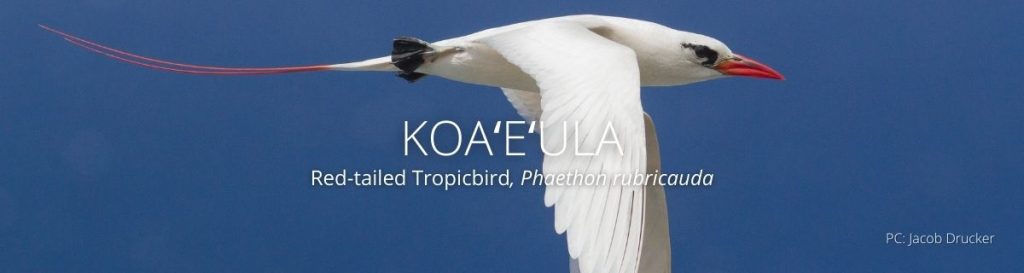This is a horizontally elongated, vibrant photo of a "Red-tailed Tropicbird" (Phaethon rubricauda) captured mid-flight, with a background of a deep blue sky. The sleek bird dominates the upper center of the frame, elegantly showcasing its mostly white plumage. Its streamlined body features a gently arched back leading to a rounded head, which faces the right side of the image. The bird's beak is vividly red, subtly sloping downward, complemented by a distinct black outline around its eyes. 

Noteworthy details include its black feet, reinforced by a small, black fin-like structure at its tail's base. The most striking characteristic is the long, split, red tail which gracefully curves upwards towards the end, extending almost from the middle of the picture to the left. The bird's wings are captured in a downward flap position, displaying the long, white feathers of the tips.

White text overlays the scene: "Koa'e 'ula" in bold, capital letters, translates to "Red-tailed Tropicbird," followed by "Phaethon rubricauda" in smaller print. The image is credited in the bottom right corner to "P.C. Jacob Drucker."